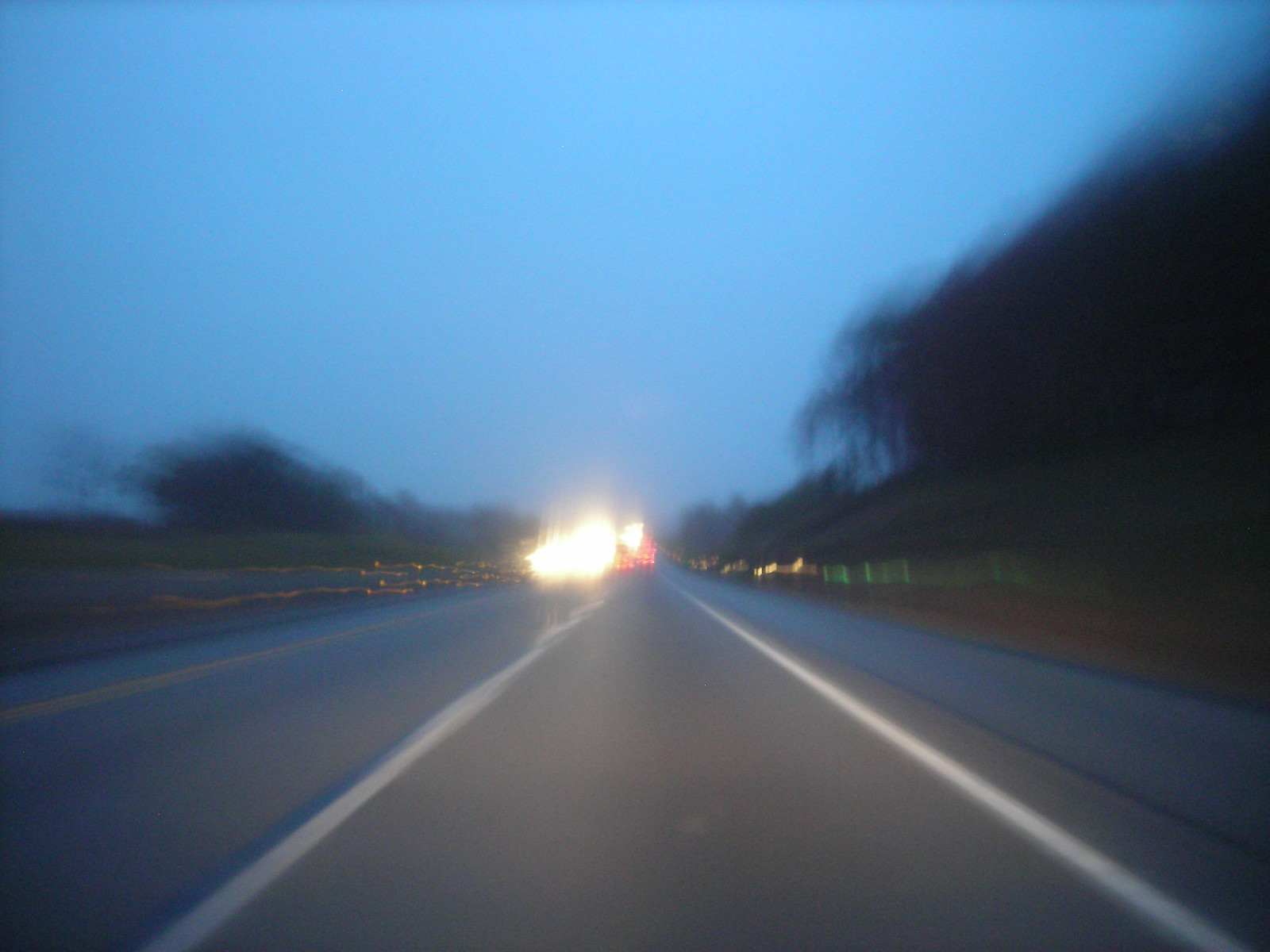A heavily blurred photograph captures a two-lane highway at dusk. The gray concrete road features a central white line dividing the lanes, with an additional white line on the right and a yellow line to the left. The shoulder, composed of darker, bumpier tar concrete, lines the edge of the highway. On either side of the road, overgrown green grass and sparse wooded areas are visible. The left side of the image shows the blurred headlights of an oncoming vehicle. Guardrails with yellow reflectors are faintly discernible along the road. The sky, a deepening dark blue, suggests the approaching twilight, with the shadows of trees stretching softly into the distance. The viewpoint mimics that of a driver’s perspective, adding to the overall sense of motion and blurriness in the photo.